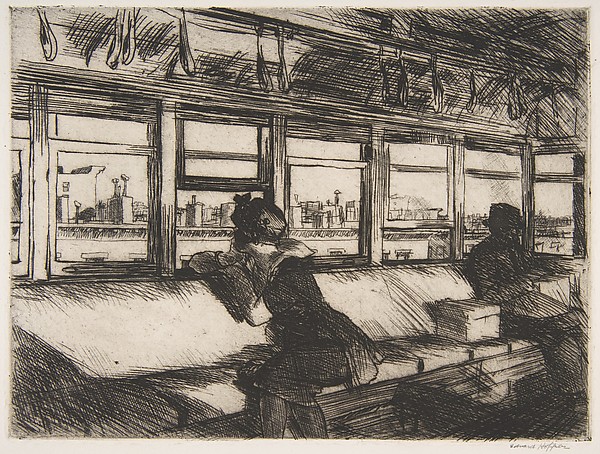This is a meticulously crafted black pencil sketch, framed by a thin white border with an illegible signature in the lower right corner. The sketch features a scene inside what appears to be a city bus or train. A woman, positioned on the left side of a long bench that spans from left to right, is gazing intently out of an open window at a cityscape filled with tall buildings. She rests her chin on her right hand, with her left hand holding onto the back of the bench, her legs crossed, and dressed in a skirt, short-sleeved jacket, and hat. On the right side, there is a man cloaked in shadow, holding a box and sitting next to another box, facing forward with a straight-ahead stare. Above the pair, rows of windows reveal the urban landscape outside, and numerous hand straps hang from the ceiling, suggesting a mode of public transportation. The entire composition has an extremely scratchy texture, achieved through vigorous back-and-forth pencil strokes to create detailed shadows and textures.